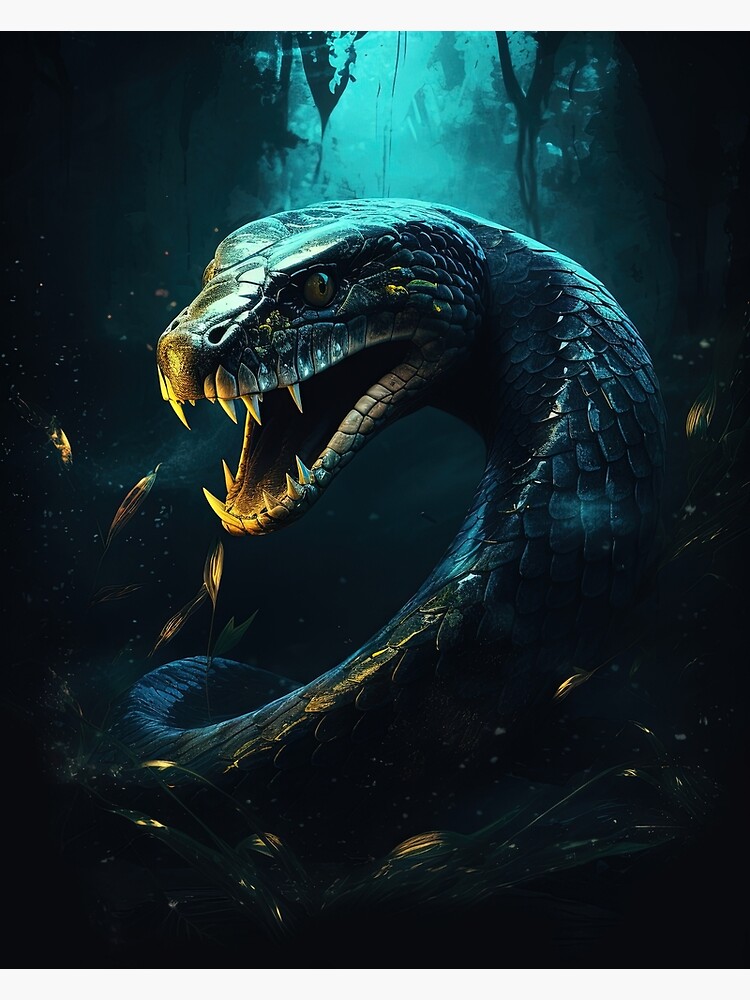The image depicts a highly detailed and mystical drawing of a large snake with its body curled into a backwards C shape. The snake's mouth is wide open, showcasing its exceptionally sharp teeth. There's a golden-yellow light illuminating its head and teeth, contrasting with its bluish-grayish-green scales. The background is very dark, adding to the eerie, ominous feel, with some aqua light blue tones above the snake and indistinct, shadowy forms that may be trees flanking either side. The snake, which appears ready to strike, dominates the scene, with the rest of its thick, substantial body trailing off into the darkness. Flecks of light sporadically pierce the gloom, enhancing the mystical atmosphere surrounding the fearsome creature.